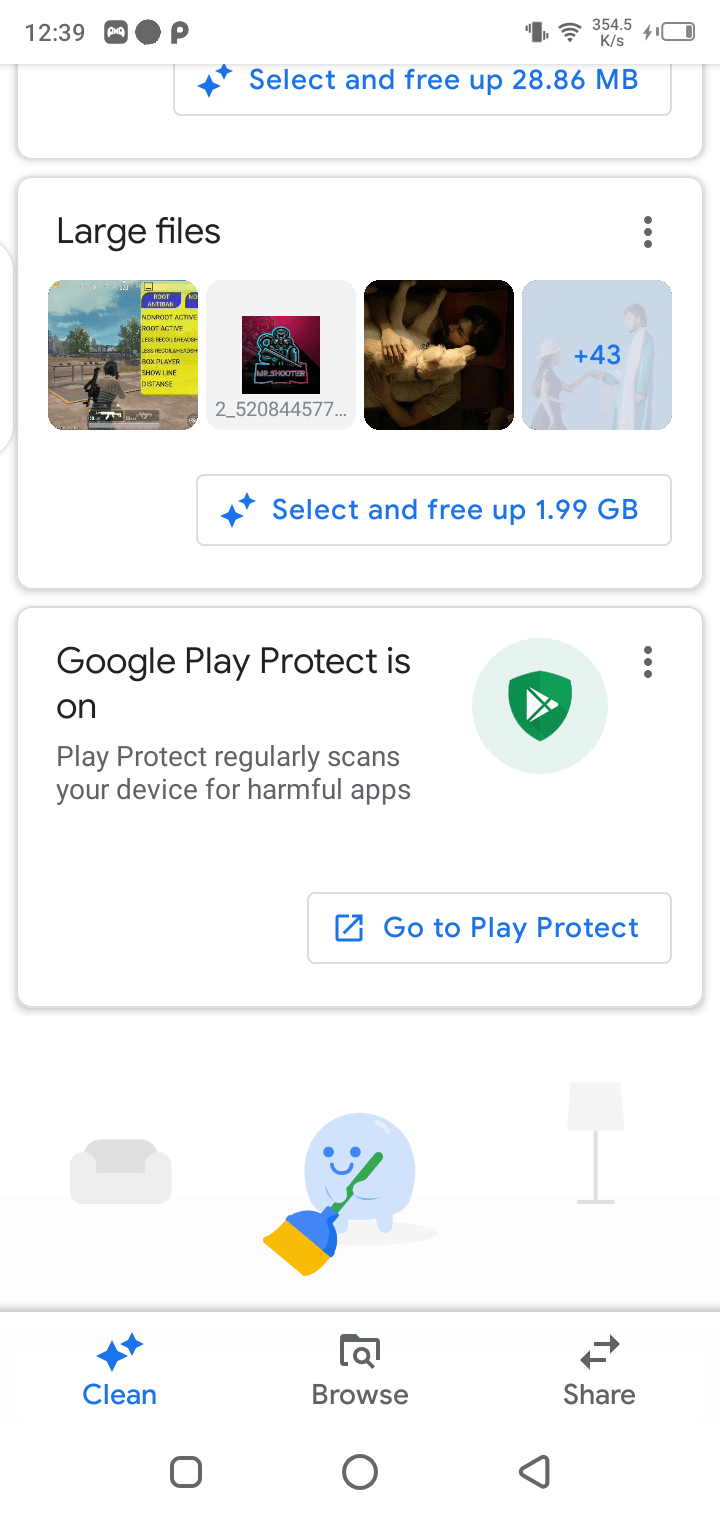This is a vertically oriented rectangle image, captured from a smartphone. The screenshot, with a predominantly white background, features the phone's status bar at the top. On the upper left-hand side, the time is displayed as 12:39, with three small icons next to it. Moving to the right, there are icons indicating the phone is on vibrate, connected to Wi-Fi, displaying download speed, and showing a battery being charged.

A thin gray borderline separates this status bar from the content below, which is organized into three distinct sections. The first section is titled "Large files" and features thumbnails of three files, with an additional notation of "43 more" on the right. Below this is a prompt to "Select and free up 1.9 GB."

The second section indicates "Google Play Protect is on," explaining that Play Protect regularly scans the device for harmful apps, with a link to "Go to Play Protect."

The final section features an image of a couch, a circular icon with a smiley face, and a broom. This section is positioned at the bottom of the image.